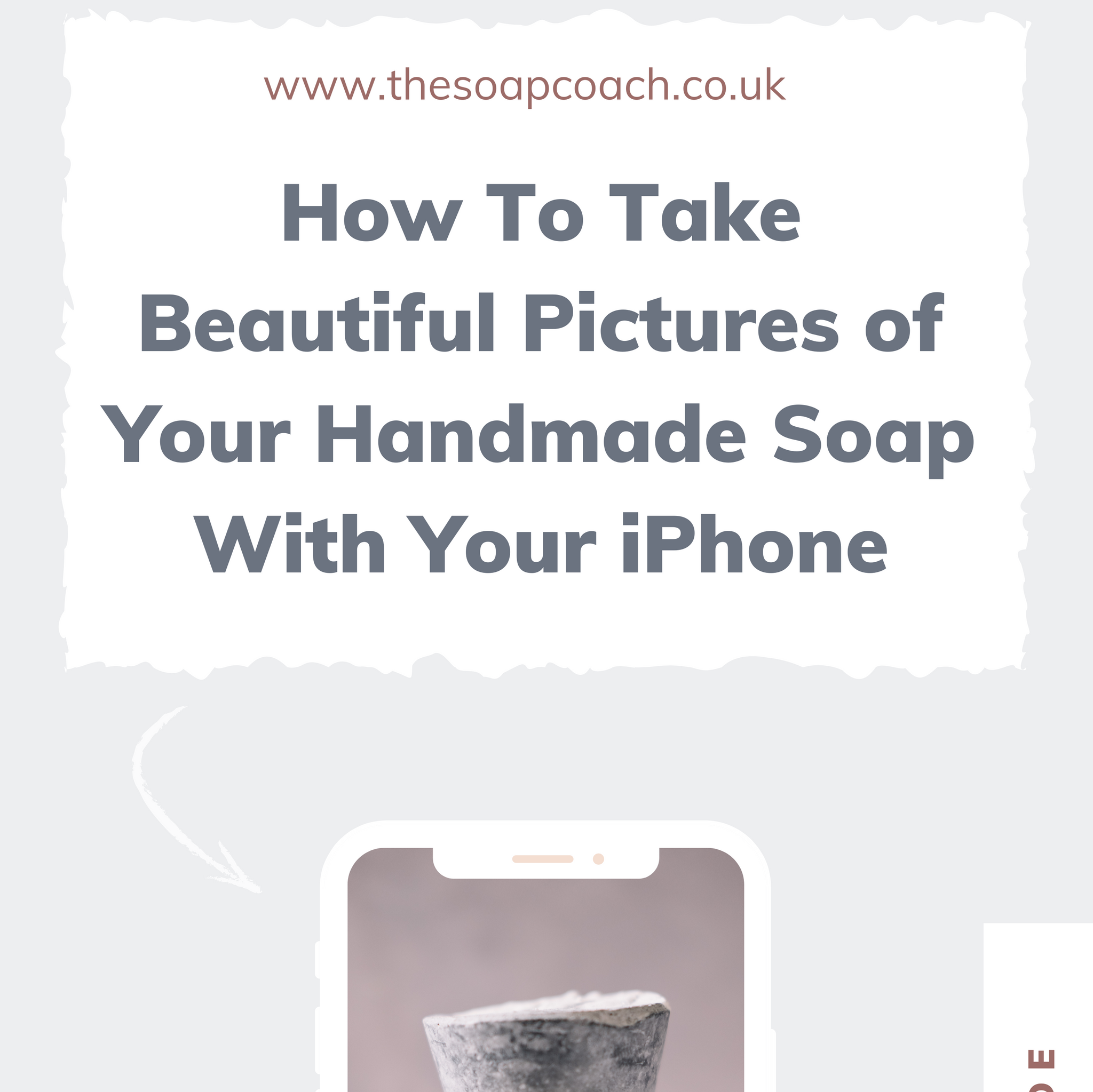The image is a detailed leaflet set against a light gray background. At the top, there is a square with jagged edges, resembling torn paper, which includes the text "www.thesoapcoach.co.uk" in light purple letters. Below this, in black and gray text, is the title: "How to take beautiful pictures of your handmade soap with your iPhone," presented with each word's first letter capitalized. A white arrow curves downward from the title to the bottom part of the leaflet, pointing at a depiction of a white-edged iPhone with a light purple screen. The top of the phone bears a distinctive pink dot and line where the camera would typically be. Beneath the phone illustration is a circular gray and white object, likely representing a piece of soap.